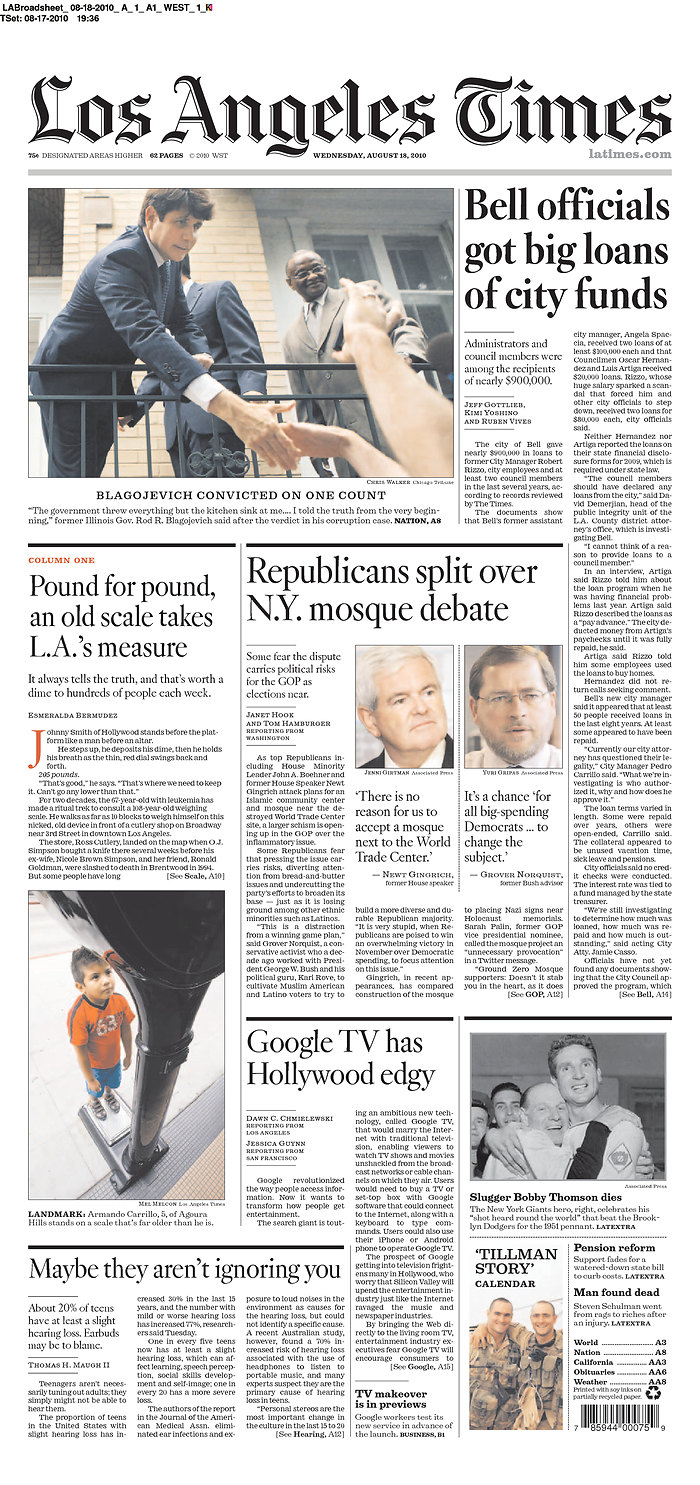The image is a close-up of the front page of the Los Angeles Times newspaper dated August 18, 2010, with the code "L.A. Broad Street 0-08-18-2010-A-1-A1-West-1" on the top left corner. The timestamp reads "08-17-2010 19:36" in military time. The Los Angeles Times title is prominently displayed in bold black.

In the main image, several political figures are depicted. A light-skinned man with brown hair, dressed in a dark gray suit and white undershirt, is seen shaking hands with people. Behind him, another individual is walking in a lighter gray suit. There is an African American man wearing a tan suit, glasses, a brown tie, and a white undershirt who appears to be reaching out toward the crowd. They are standing next to a brown brick building with a white facade.

The headline underneath reads in bold black, "Blagojevich Convicted on One Count." Followed by a quote: "The government threw everything but the kitchen sink at me... I told the truth from the very beginning," attributed to former Illinois Governor Rod R. Blagojevich after the verdicts in his corruption case.

Additional headlines include "NATO" followed by "Bell Officials Got Big Loans of City Funds." On the left-hand side, there are stories titled "Pound for Pound: An Old Scale Takes LA's Measure," "Republicans Split Over NY Mosque Debate," "Google TV Has Hollywood Edgy," and "Maybe They Aren't Ignoring You." On the right-hand side, another headline reads "Tillman Story Calendar."